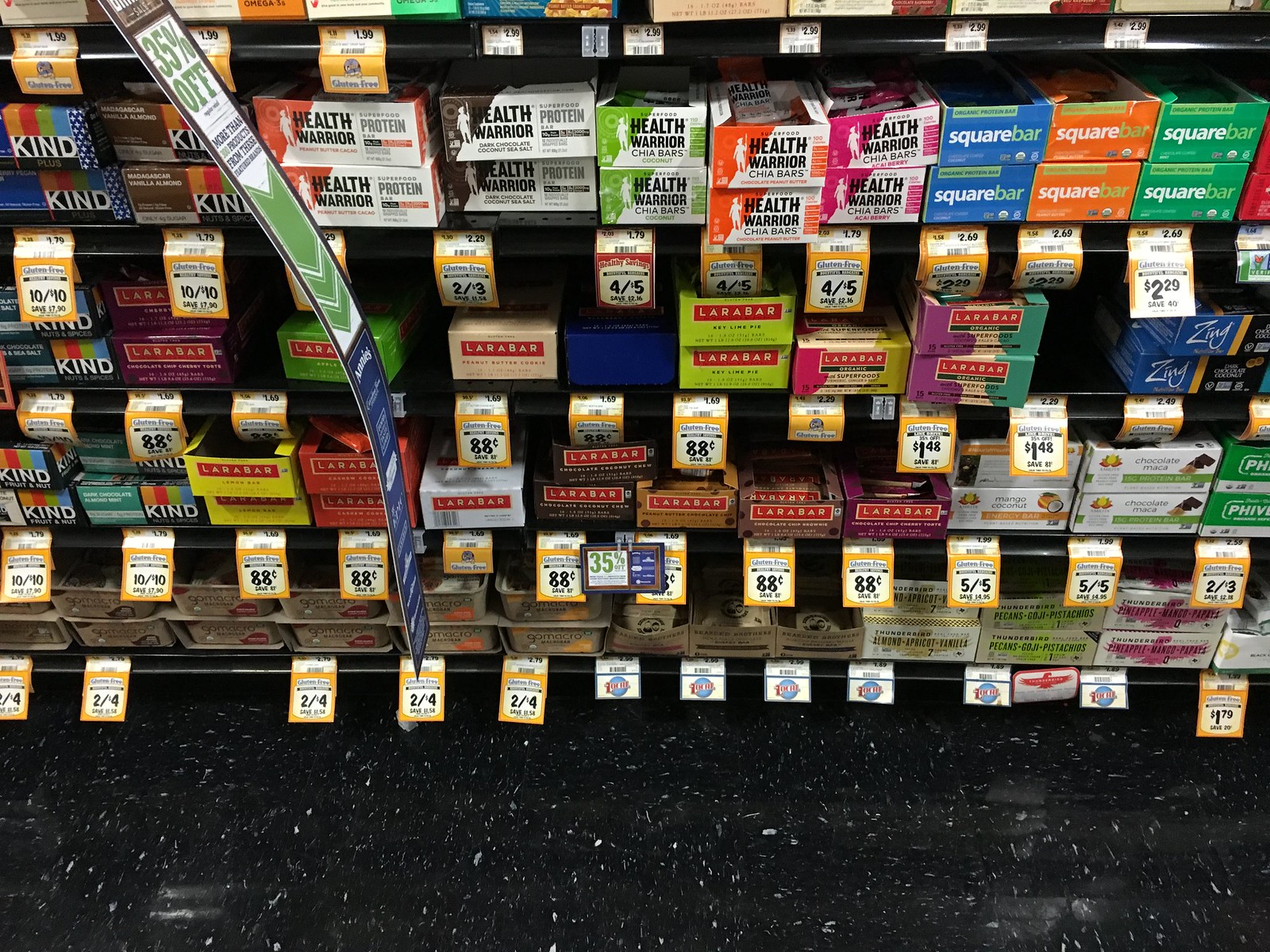This image captures the protein, energy, and health bar aisle at a bustling grocery store. The shelves are laden with an extensive assortment of brands and flavors, catering to every taste and nutritional need. There are five fully-stocked shelves, each brimming with a variety of options, many of which are marked with enticing sale tags, suggesting significant discounts across the board.

On the highest visible shelf, a multitude of brands are represented, although some products are partially obscured. Prominent among these are a generous selection of Laura Bars in flavors such as mango, coconut, chocolate, and maca protein. Other notable brands include Kind Bars, Health Warrior Protein and Chia Bars, Square Bars, and Zing Bars.

Descending to the bottom shelf, the diversity continues with brands like Go Macro and Thunderbird taking center stage. Specific flavors noted on this shelf include almond, apricot vanilla, pecan, goji, pistachio, pineapple, mango, and papaya, illustrating the wide range of exotic and traditional flavors available.

Though the specific store remains unidentified due to indistinct tags, the vibrant display of health bars showcases a microcosm of the myriad nutritional choices available to health-conscious shoppers.